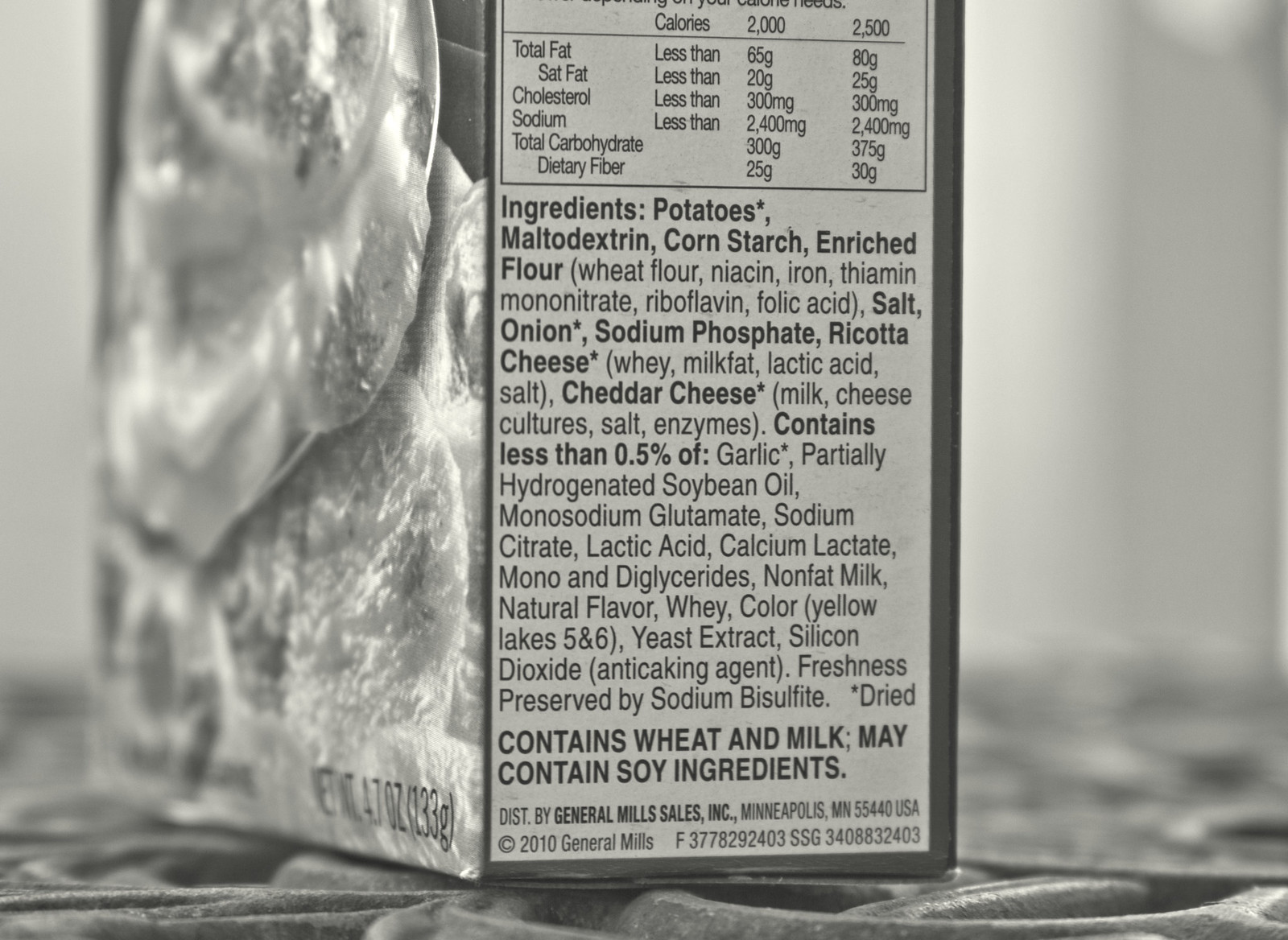This is a monochromatic photograph of a container, likely a box of powdered potatoes or a similar product, displayed on a wrought iron table. The image is black and white, highlighting the detailed text on the side of the box. The front of the container appears to feature a blurred image, possibly depicting potatoes or another type of fruit like oranges. The side of the container lists ingredients in black font against a white background, starting with potatoes, malt, oat, cornstarch, and enriched flour, which includes wheat flour, niacin, iron, thiamine mononitrate, riboflavin, and folic acid. Additional ingredients mentioned are salt, onion, sodium phosphate, potassium phosphate, ricotta cheese, whey, milk fat, lactic acid, and cheddar cheese, which contains milk and cheese cultures. The label also indicates that the product contains wheat and milk, and may contain soy ingredients. The document reveals the product's weight as 4.7 ounces and mentions that it is produced by General Mills Sales Incorporated, located in Minneapolis, Minnesota.